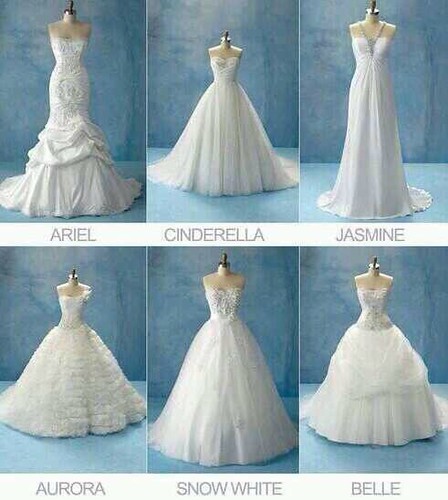This image, presented on a white background, showcases six individual photos arranged in two rows of three. Each photo depicts a headless and armless mannequin adorned in a distinct wedding dress, set against a blue background with blue flooring. These mannequins, each labeled with black text beneath their respective gowns, are named after Disney characters: Ariel (top left), Cinderella (top center), Jasmine (top right), Aurora (bottom left), Snow White (bottom center), and Belle (bottom right). The dresses are predominantly white, featuring various designs that range from puffy to off-the-shoulder and strapless styles, with some having sweetheart necklines. One of the gowns includes a halter strap design. The elegant display emphasizes the unique beauty of each wedding dress, against the soft blue backdrop that enhances their pristine white fabric.